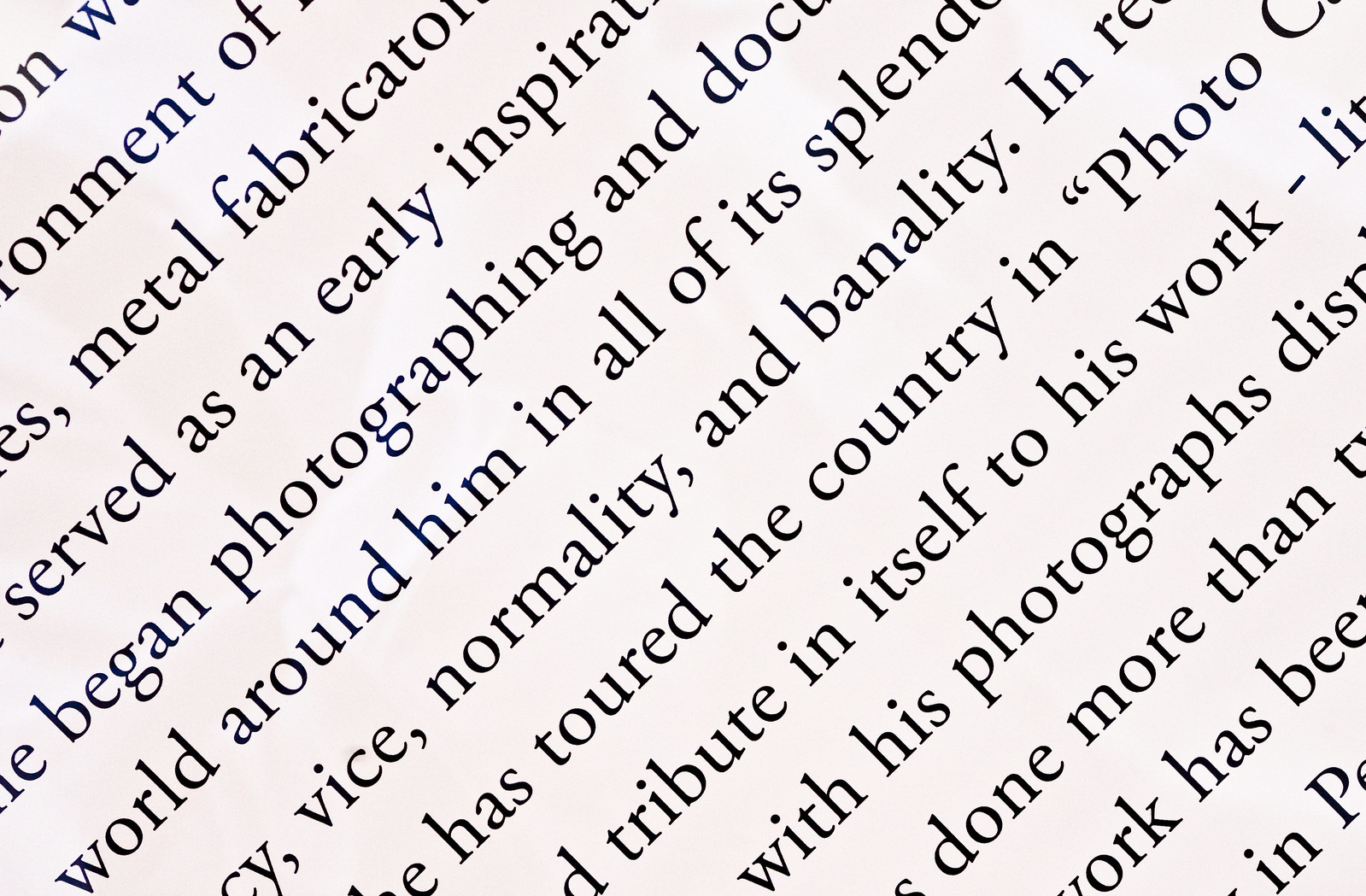This image features a square frame with a pale pink background and black diagonal text, running from the bottom left to the upper right. The text appears to come from a page of a book, detailing the work of a photographer. The sentences are cut off at the edges, making only parts of them readable. Phrases like "metal fabrication served as an early inspiration," "began photographing and documenting the world around him," and "toured the country in photo tribute" are visible. The words are slanted, suggesting the photo of the page was taken at an angle, causing some partial words in the corners and more complete sentences in the middle. Despite the truncated nature and lack of context, the text describes a photographer's career and inspirations, with mentions of exhibitions and the various themes he captures.